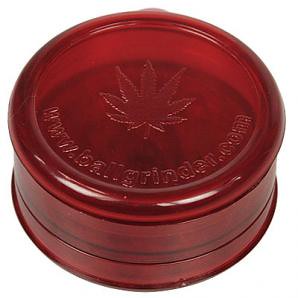The image depicts a small, circular, dark red plastic weed grinder approximately two inches tall. This grinder features a sunken center with a marijuana leaf pattern, characterized by its seven slender, pointed leaves. The transparent material allows visibility inside the object. On the rim, the text "www.ballgrinder.com" is inscribed in the same red color as the grinder. The top of the grinder appears to be removable, suggesting it can be used to store and grind marijuana buds. The top half is slightly lighter in shade compared to the darker bottom half.